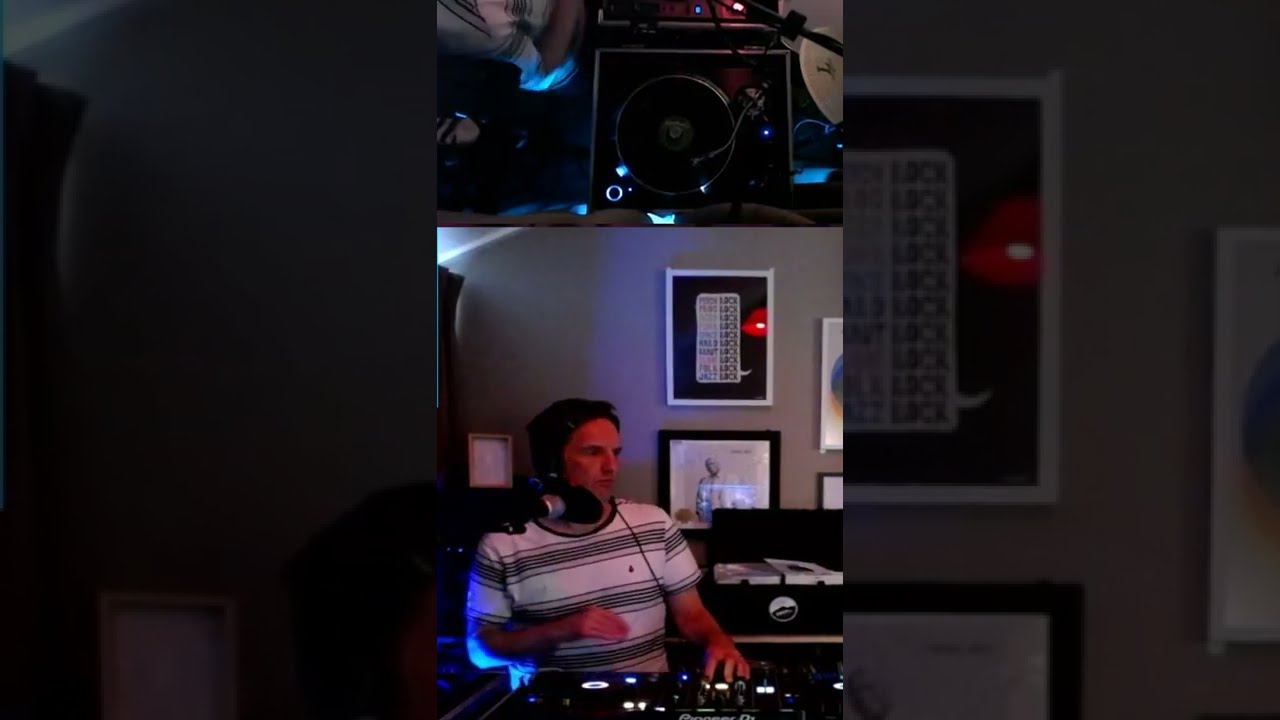The image captures a live-stream session featuring a man deejaying in what appears to be his home. The composition splits into two layers: the central focus being a vertical cell phone picture of the DJ, with a zoomed-in, faded, and darker version of the same image forming the background. The man, a white male with black hair, is wearing a white striped t-shirt and headphones with a cord trailing down his left side. He is actively engaged with his DJ equipment; his left hand is on the turntable or mixing board, while his right hand is raised horizontally. Notable details include the silver tone arm of the turntable resting on a black vinyl record, and a microphone positioned close to his mouth. Blue lighting subtly illuminates the scene. The setting appears to be a home office, identifiable by a gray drywall background adorned with framed artwork. Additionally, there is a separate top-down view focusing on the turntables, reinforcing the DJ's involvement in the live session.